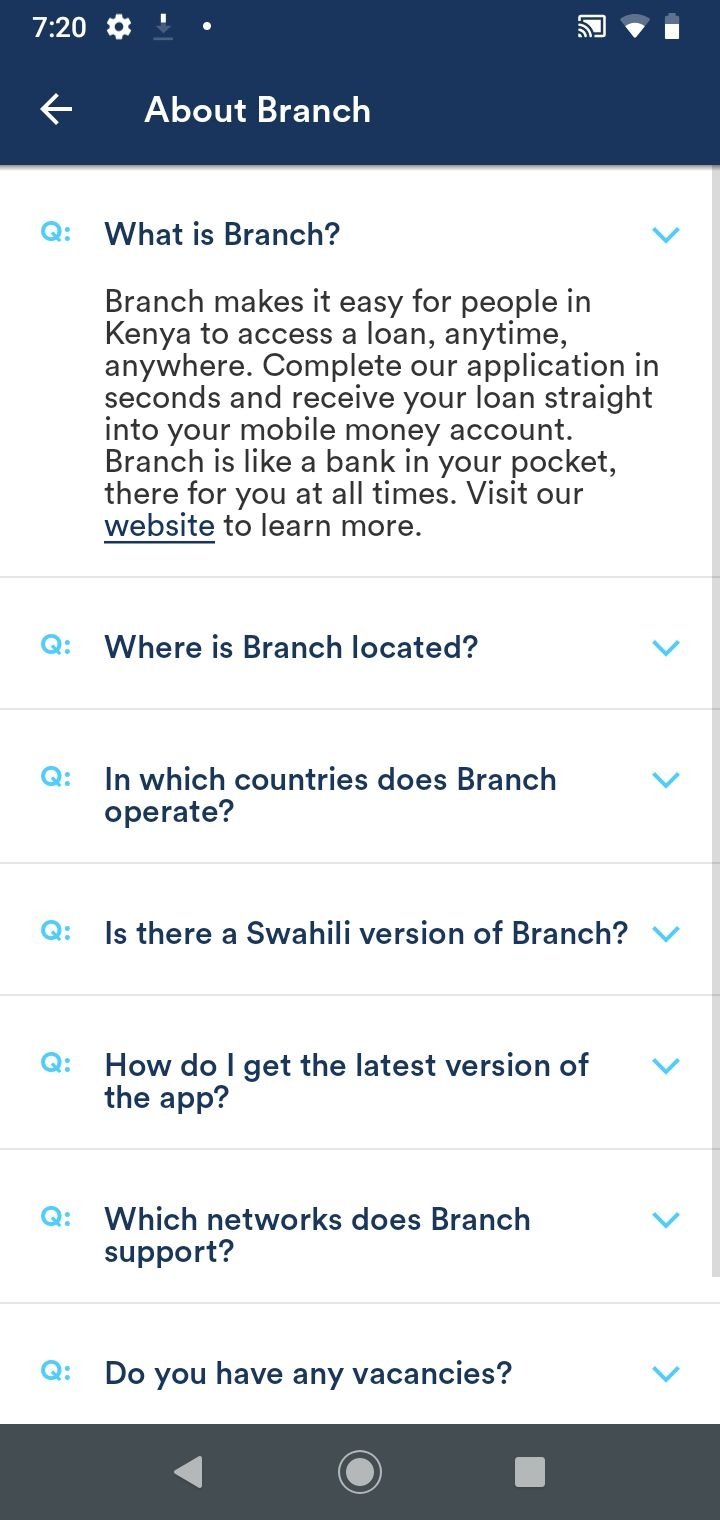This screenshot, taken from a smartphone, captures a detailed interface of a financial services app. In the top left corner, the time displayed is 7:20, accompanied by several status icons. On the upper right side, additional symbols, including an internet icon and a padlock symbol, are visible, all set against a dark background.

Below this, there's a blue header featuring a left-pointing arrow and the text "About Branch". The remainder of the screen has a white background with a prominent block of text. A blue question (Q) icon poses the query, "What is Branch?", followed by an informative answer. The text explains that Branch provides easy access to loans for people in Kenya, allowing users to apply within seconds and receive funds directly to their mobile money accounts. Branch is described as a "bank in your pocket," always available for users, with an invitation to visit their website for additional information.

Further down, there are more interactive Q&A lines:
- "Where is Branch located?" with a down arrow indicating more information on click.
- "In which countries does Branch operate?" also accompanied by a down arrow.
- "Is there a Swahili version of Branch?"
- "How do I get the latest version of the app?"
- "Which networks does Branch support?"
- "Do you have any vacancies?"

At the bottom of the screenshot, a dark bar houses navigation icons—a white left-pointing triangle, a circle with a dot in the center, and a white square. Overall, the image showcases an informative section of a mobile app designed to help Kenyan users access financial services easily.